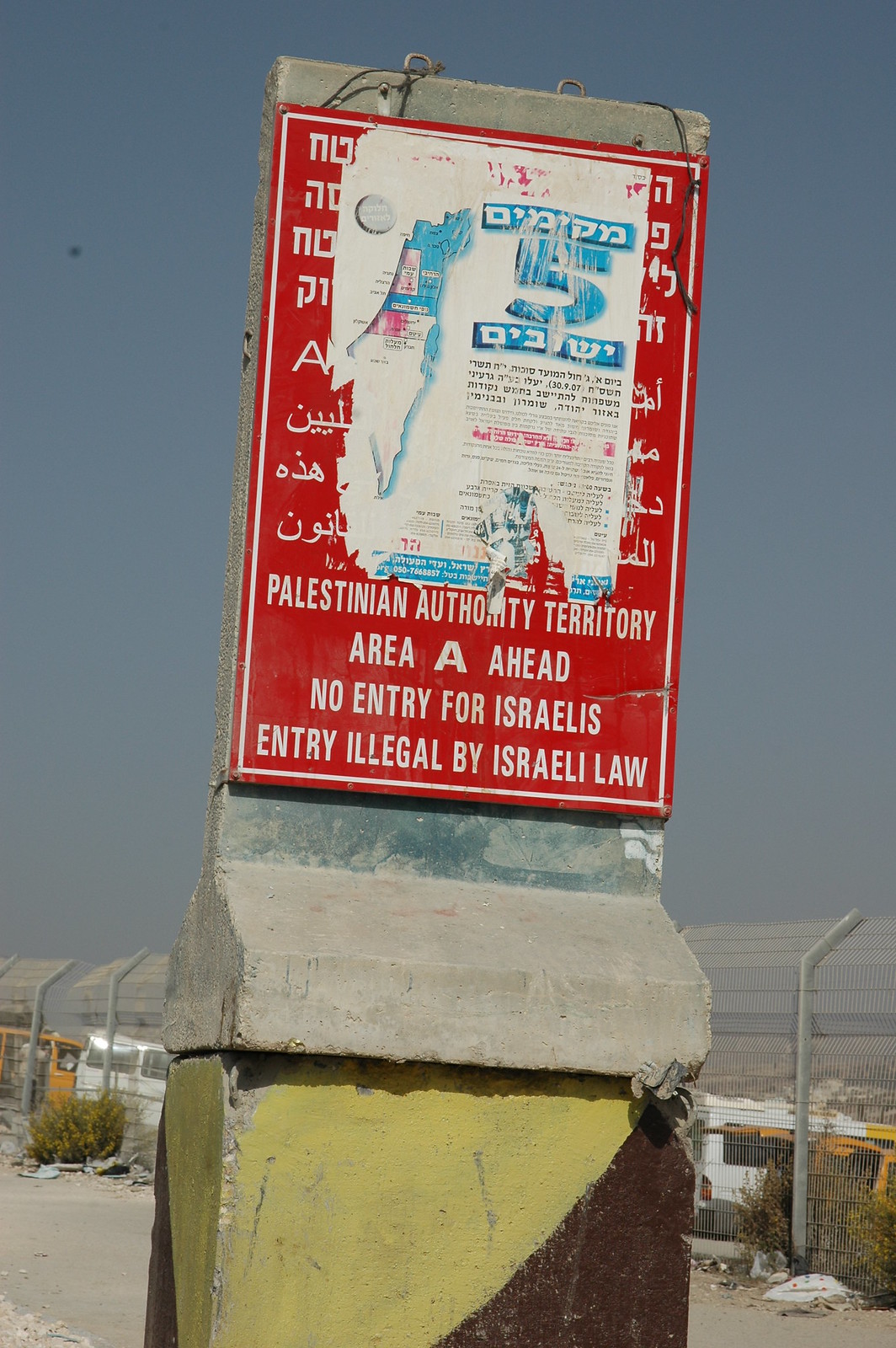The image depicts a no-entry sign supported by a uniquely shaped, multi-colored concrete pillar. The pillar consists of a yellow section at the bottom, a brownish side, and a grey top, which is somewhat triangular in form. On top of this pillar rests a red sign with prominent white text that reads: "Palestinian Authority Territory. Area A ahead. No entry for Israelis. Entry illegal by Israeli law." The sign includes additional texts in different languages, likely European and Arabic, with portions partially obscured by a torn white paper that displays the number "5" encased in blue bars above and below. Behind this setup, a tall, grey fence curves outward at its top and spans across the background. To the right of the yellow block, two white vans are parked, while on the left, two yellow vans are stationed. A person dressed in a tan jacket and blue jeans stands in the doorway of one of the vans on the left. The overall backdrop includes a hazy, sunny sky.